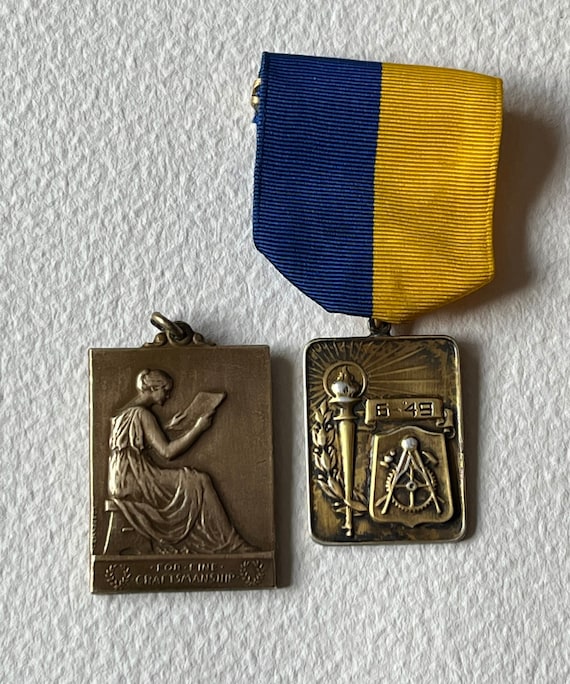The photograph depicts two bronze-colored military-type medals side by side. The medal on the left, which is slightly larger, features an image of a seated woman in an ancient-style gown, reading from a piece of paper or parchment. Below the woman, the inscription "For Fine Craftsmanship" is engraved, flanked by two olive branches. The medal on the right, which is slightly smaller, is attached to a folded blue and yellow ribbon. It displays an image of an Olympic torch emitting radiating light, encircled by a flower or vine, and includes the number "6-49" and the symbols of a compass, square, gear, and a hammer engraved onto it.